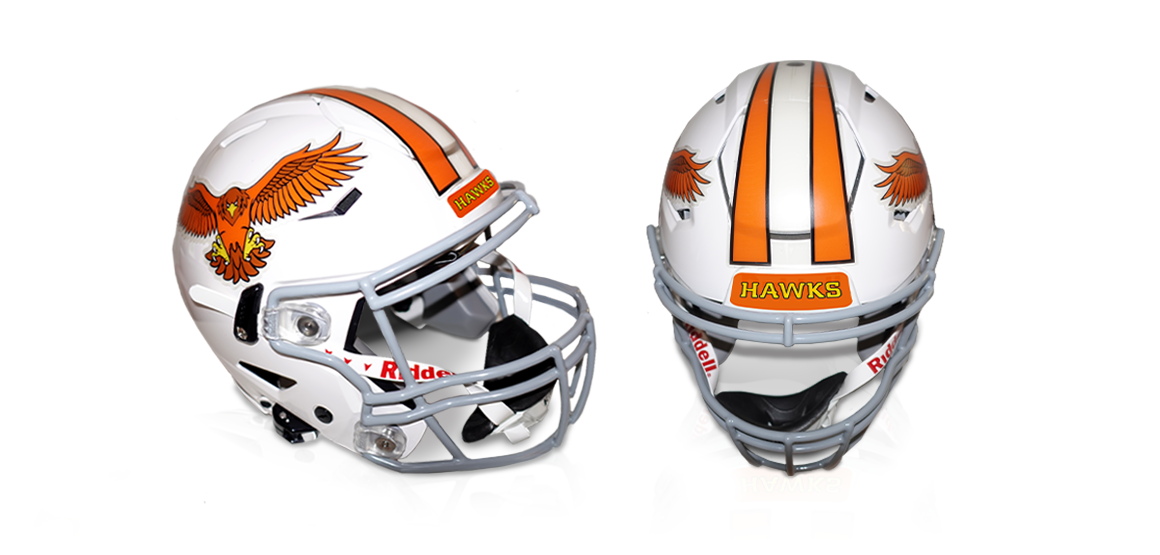This is an artistic rendering of a football helmet, displayed from both side and front views. The predominantly white helmet features bold design elements, including two orange stripes running from the top to the back. On each side of the helmet is a dynamic image of an orange hawk, wings spread wide as if in attack, with yellow talons and beak. The front view showcases the team name, "Hawks," written in yellow letters outlined in orange, on a red rectangular background located just above the face mask. The face mask is a thick, gray-painted steel frame, complemented by a red "Riddell" logo on the white chin strap. The detailed views highlight both the side profile with the aggressive hawk imagery and the front with the prominent team name, making the helmet a striking piece of sports equipment.